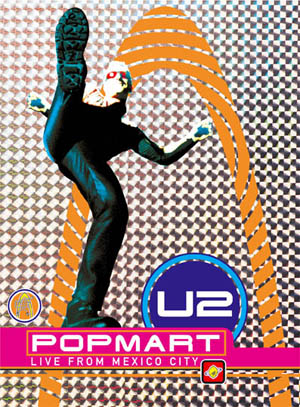This image is a promotional poster for a U2 concert. The backdrop features an interlaced black and white checkerboard pattern, which resembles a brick design. At the center is a large, domed orange or yellow shape, almost like a halo. Bono, the lead singer of U2, is prominently depicted as a cartoonish or blended illustration. He is dressed in all black – wearing black leather pants, black boots, and a tight black turtleneck shirt. His hair is white-bleached, and he sports his iconic red sunglasses. Bono is striking a dynamic pose, balancing on his left leg while his right leg is kicked up high, revealing the sole of his right shoe. A blue circle on the poster displays the text "U2" in white. Below this, in a pink banner, the white lettering reads "Pop Mart, live from Mexico City," indicating that this is an advertisement for U2's Pop Mart tour, likely from the late 1990s.